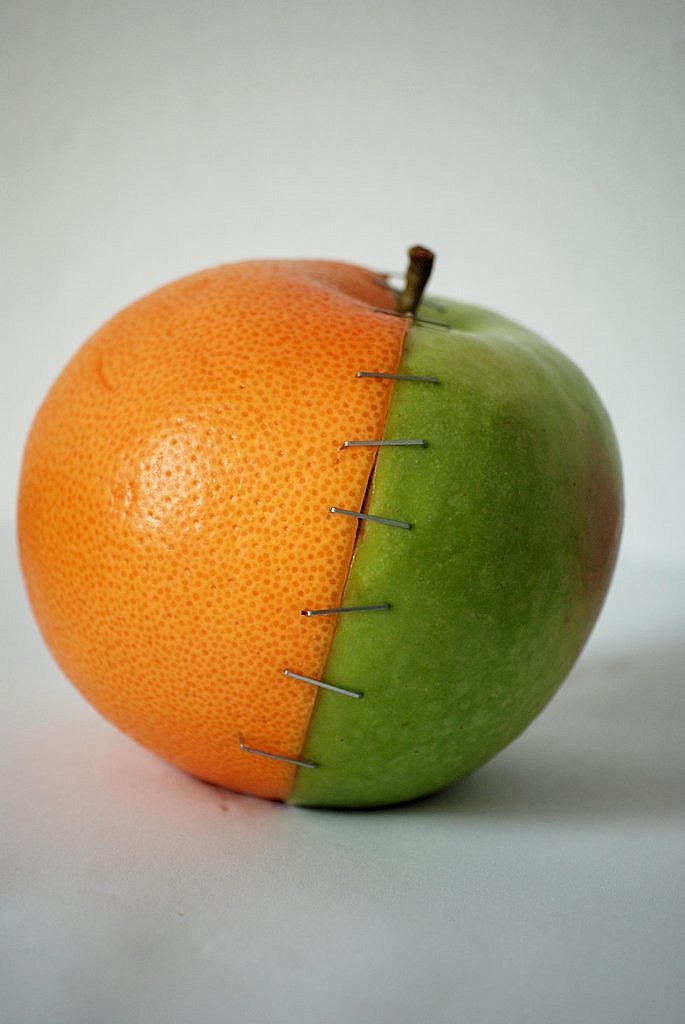This photographic image showcases a fascinating hybrid fruit against a gray indoor background. The composition consists of one half of an orange seamlessly joined with one half of a green apple, which has a touch of red on the outer edge. The fruits are melded together using six silver staples, positioned mostly horizontally with a few angled, securing the pieces firmly. The apple’s stem remains intact, protruding from the top. The orange half, situated on the left, exhibits a glistening shine due to the reflected light and features a small nick as if from a fingernail. The combined fruit leans slightly to the right, creating a subtle yet intriguing tilt. Shadows cast on the gray wall further enrich the visual depth of the composition, which remains free of any text elements, allowing the unique fruit to captivate the viewer’s full attention.